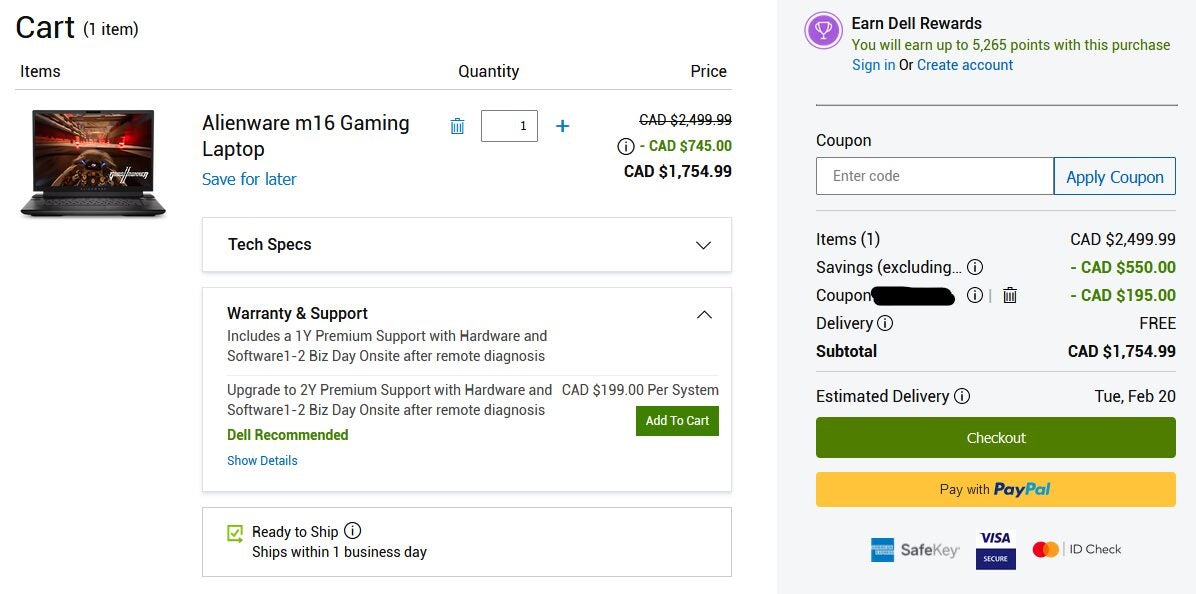The photograph is divided into two distinct sections. The left-hand side features a predominantly white background. At the top, the word "Cart" is displayed in bold black text, followed by "1 item" in parentheses, also in black. Directly below, the header is labeled "Items," and adjacent to it, "Quantity" and "Price" are noted in black lettering. A thin horizontal line separates this header from the content below.

Central to the left section is the featured item: an Alienware M16 gaming laptop, which is presented in black text next to an image of a sleek black laptop. A blue-colored trash can icon is visible beside it. The quantity of the item is indicated within a white box outlined in black, showing "1" with a plus sign for adjustment. Beneath this is an option to "Save for later."

Regarding the price details, the original price is listed as CAD $2,499.99, which is struck through. A green reduction of CAD $745.00 is prominently noted, resulting in a final price of CAD $1,754.99. Additional information further elaborates on the item's specifications: "Tech Specs," "Warranty and Support," which includes one year of premium support covering both hardware and software, with a promise of reaching the site within one to two business days following remote diagnosis procedures. Shipping is prompt, as the item is "Ready to ship" and "Ships within one day."

The right-hand section of the image has a gray background featuring the final price and checkout options. Customers are provided the opportunity to check out and may utilize various payment methods, including PayPal, Micro Express, Seiki, Visa Secure, MasterCard, and ID check.

The overall impression is a meticulously organized shopping cart overview for an Alienware M16 gaming laptop, emphasizing detailed pricing adjustments, support information, and a variety of payment options to facilitate a straightforward purchasing experience.